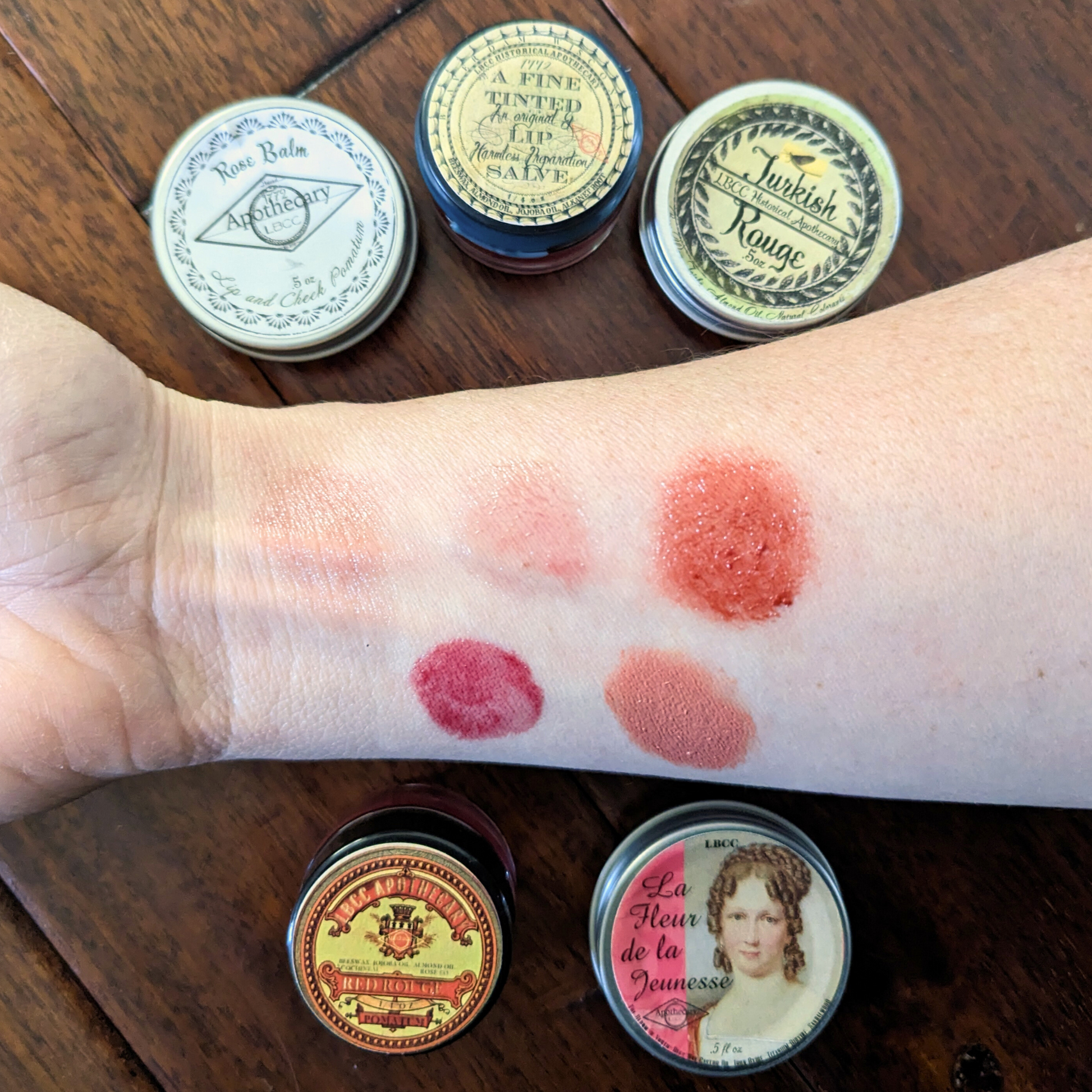The image showcases a light-skinned arm resting on a brown wooden surface, with the palm partially visible and the wrist positioned midway up the forearm. The arm is oriented left to right, with the palm on the left side of the frame. Displayed on the wrist are five different splotches of makeup, ranging from very light pink to dark maroon red. These colors represent various shades of rouge, and each is associated with a small, antique-looking tin pot shown at the bottom of the image. The tins have circular lids adorned with different labels and designs. The top row includes a white tin with blue writing labeled "Rose Balm Apothecary," a beige tin labeled "A Fine Tinted Lip Salve, 1772," and another tin labeled "Turkish Rouge." The bottom row features a tin labeled "Red Rouge" and another adorned with an image of an old-fashioned lady with ringlets, captioned "La Fleur de la Jeunesse." Each label indicates the unique type of rouge in the pots, reflecting the vintage styling of the containers.